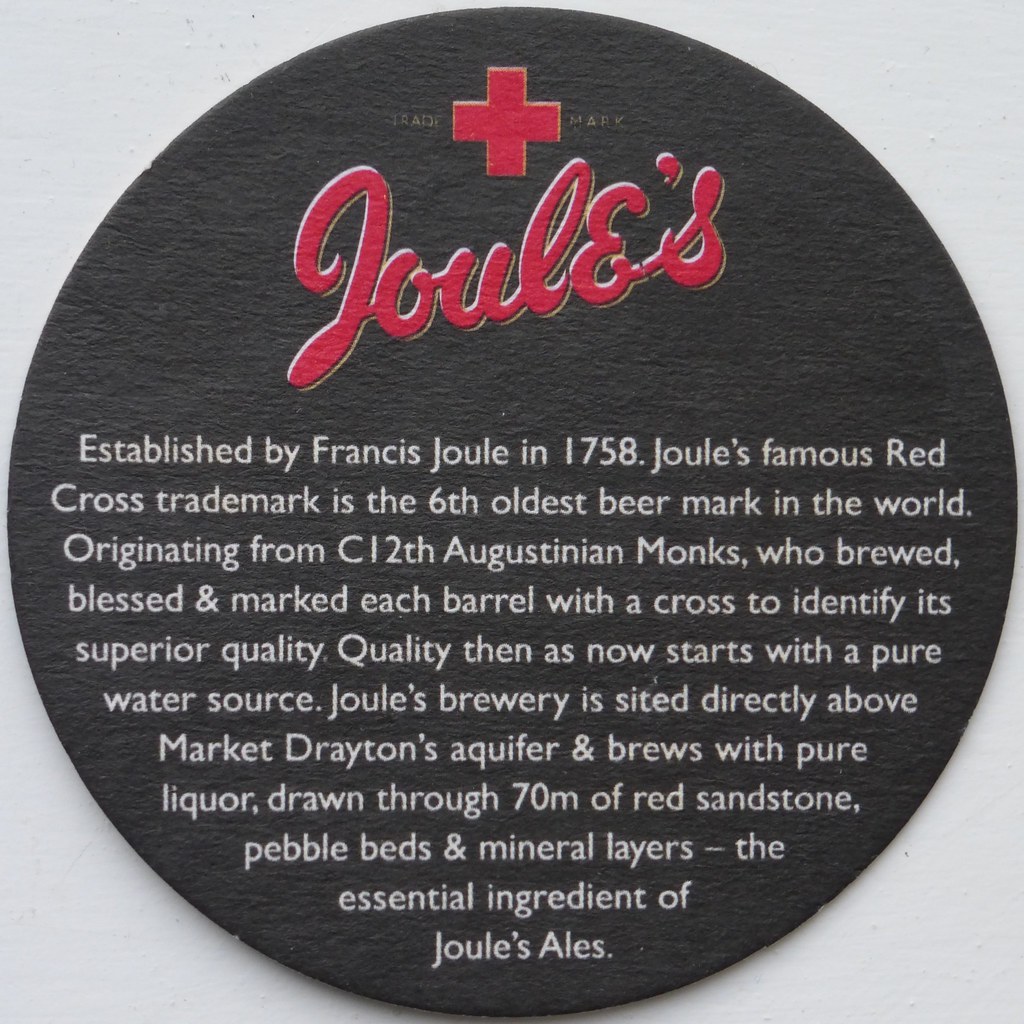This square-shaped image features a central black circle with detailed inscriptions. At the top of the circle is a red plus sign, flanked by the words "Trade" and "Mark" in gold. Directly beneath this, "Joules" appears in red cursive. Below, in white text, the plaque reads: "Established by Francis Joules in 1758, Joules' famous red cross trademark is the 6th oldest beer mark in the world, originating from 12th-century Augustinian monks who brewed, blessed, and marked each barrel with a cross to identify its superior quality. Quality then, as now, starts with a pure water source. Joules Brewery is sited directly above Market Drayton's aquifers and brews with pure liquor drawn through 70 meters of red sandstone, pebble beds, and mineral layers, the essential ingredient of Joules' ales." The image's background is light blue, creating a sharp contrast against the black and colored elements. The overall presentation suggests this could be a digital photograph of a plaque, possibly designed to resemble a beer coaster.